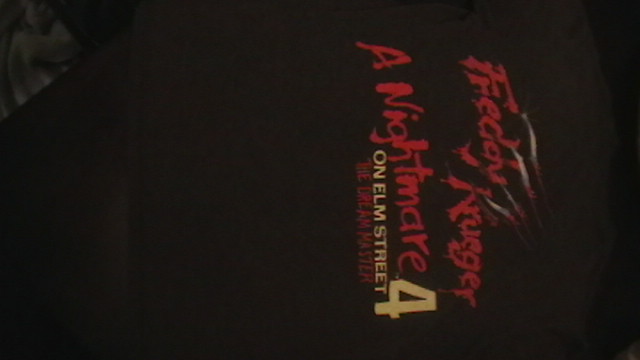This image appears to be a slightly rotated photograph, possibly taken at night, of a dark, grainy flyer or poster. The poster prominently features the text "Freddy Krueger" in a red, blood-like font, evoking a sense of horror. From the letters of the name protrude claw-like hands, scratched out in gray with hints of red. Beneath this, "A Nightmare on Elm Street 4" is written, with "A Nightmare" and "The Dream Master" also in red, smudgy text, while "On Elm Street 4" is in a crisp, beige-yellow font. The background is entirely black, adding to the eerie and ominous atmosphere, which emphasizes the horror theme of the film "A Nightmare on Elm Street 4: The Dream Master."